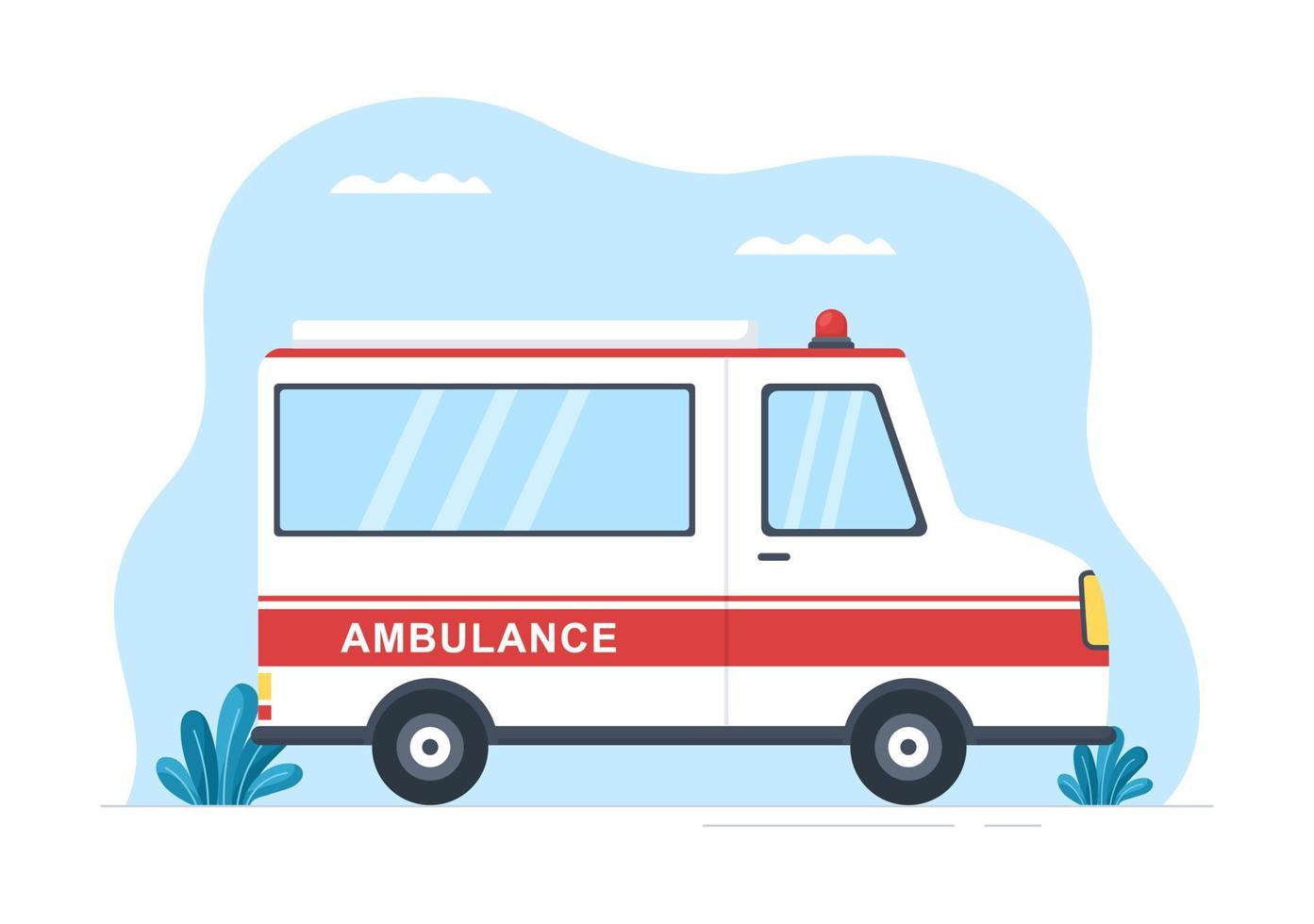The image is a bright and clear digital drawing of an ambulance. The ambulance is primarily white with a prominent red stripe running across its side, which features the word "AMBULANCE" in bold, white capital letters. It has large blue windows and a distinctive red siren on its roof. The vehicle's wheels are depicted with black tires and intricate gray, white, and black detailing inside. The scene is set against a bright blue sky with a couple of white clouds floating above. Flanking the ambulance are two bluish-green plants, one at the front and one at the rear. The overall style of the image is simple and cartoonish, with a clean and uncluttered look, including a yellow headlight at the front of the ambulance.